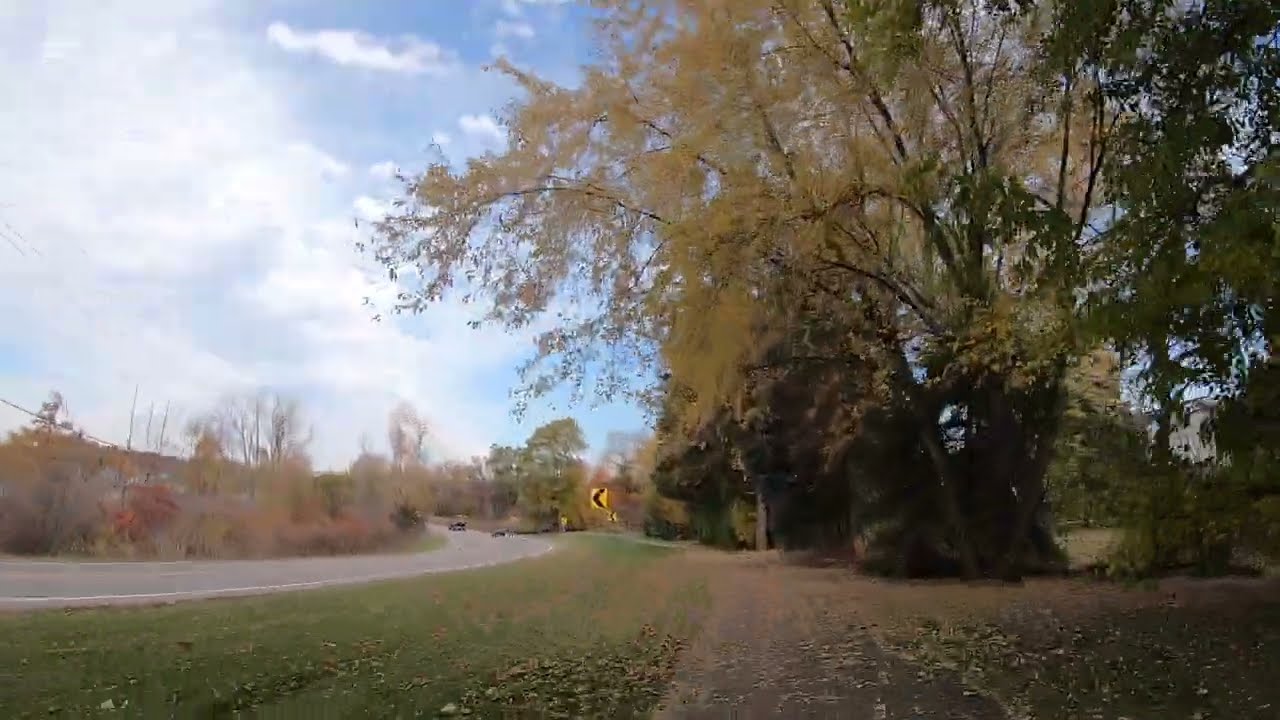This photograph captures a slightly blurry outdoor scene featuring a curved road that starts from the left and bends to the left, with two cars visible on it. On the left side of the road, the ground is predominantly covered with dry grass, small plants, and brushy shrubbery. The right side of the road showcases a gradually transitioning landscape: beginning with green grass, followed by some yellow and black signboards, and eventually leading into an area of dense trees. These trees display a mixture of green and yellow leaves, suggesting a seasonal change, possibly to autumn. Some trees on the right show fully yellow foliage, while others have leaves that are partly turned or have already fallen. The sky above is a vivid blue, dotted with white clouds, adding to the overall ambiance of the scene.